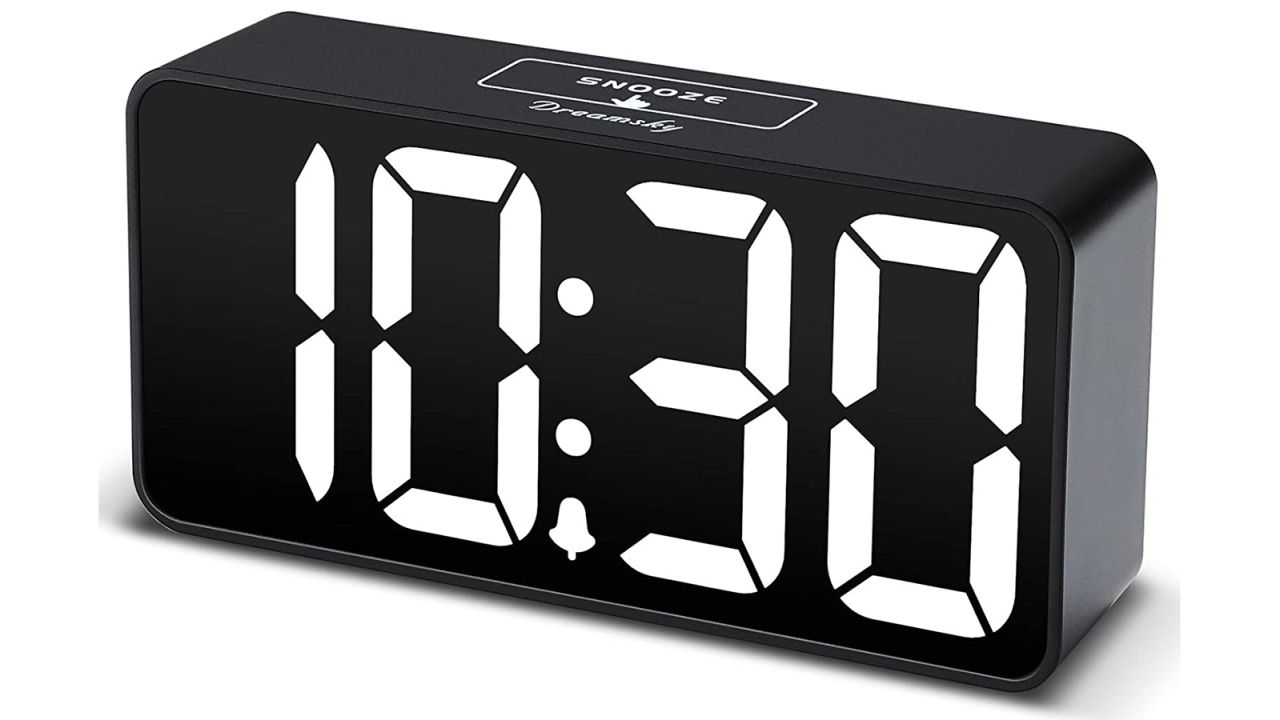The image displays a sleek, black digital alarm clock with a smooth, polished surface and rounded corners. The clock prominently shows the time as 10:30 in a cream-colored, fairly blocky font, giving the impression that the numbers are etched onto its face. At the top of the clock, surrounded by a white rectangular border, is the word "Snooze" accompanied by a small white hand illustration pointing towards it. Just below this, the brand name "Dreamly" is inscribed. An icon of a small alarm bell between the numbers indicates that the alarm is set. The clock appears to be a thin, black plastic device, possibly battery-powered, and lacks noticeable cords.